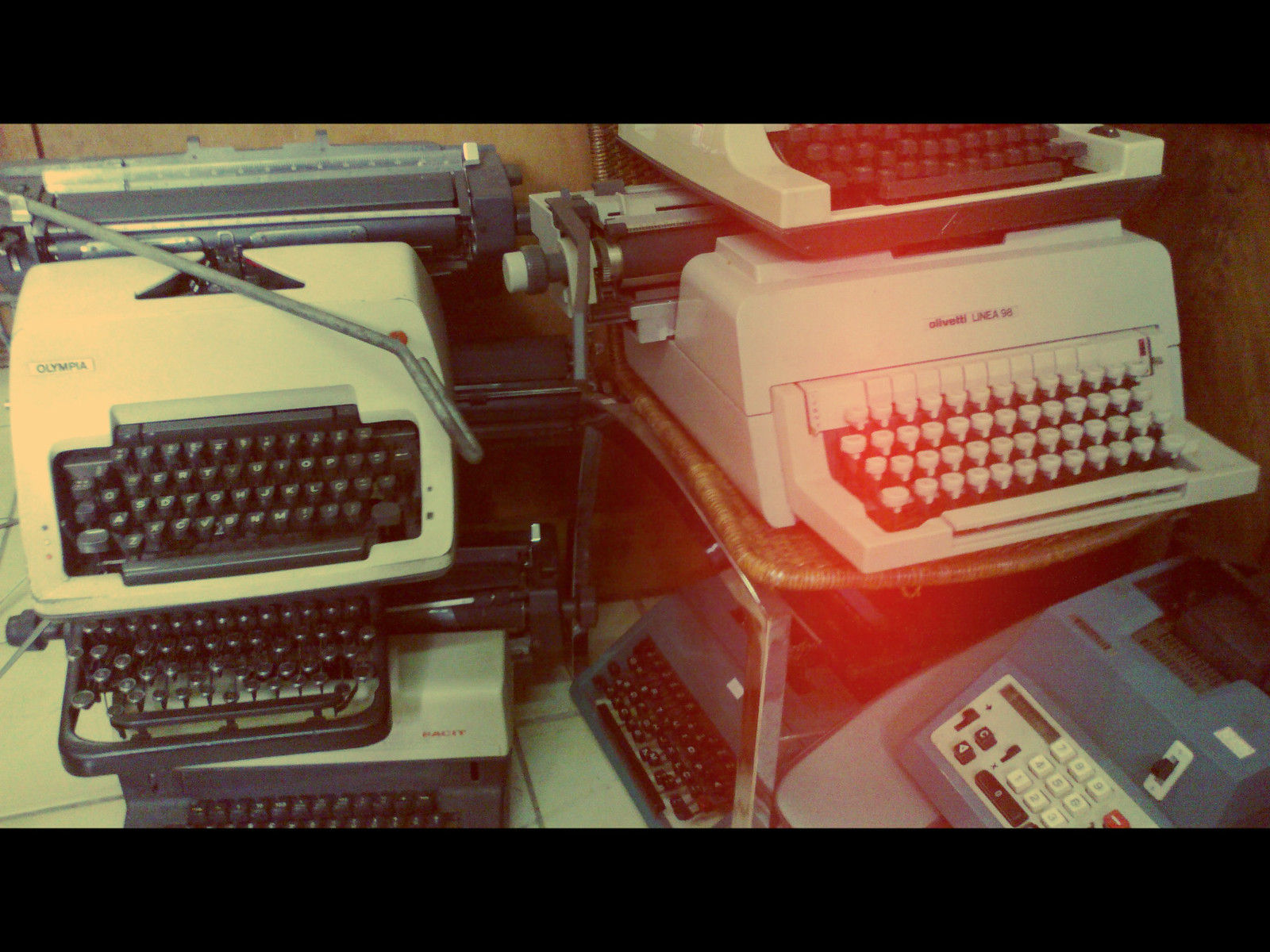The photograph features a chaotic stack of vintage and retro typewriters alongside an adding machine, all arranged haphazardly on a white tile floor. On the left side, an Olympia manual typewriter is prominently displayed, with a very old black typewriter below it, showcasing exposed keys. Further down, an electric typewriter rests at the bottom of the stack. On the right side, a juxtaposition of an electric typewriter atop a manual Olivetti typewriter captures attention, while a grayish-green adding machine sits at the bottom right. This adding machine is particularly notable for its six white numbered keys, a black zero key, and a couple of function keys accentuated by a sliding switch. The entire setup suggests a cluttered storage area or second-hand store, where these historical pieces, ranging from the 70s or 80s, appear neglected and undervalued, possibly awaiting a fate where they may never be used or sold again.